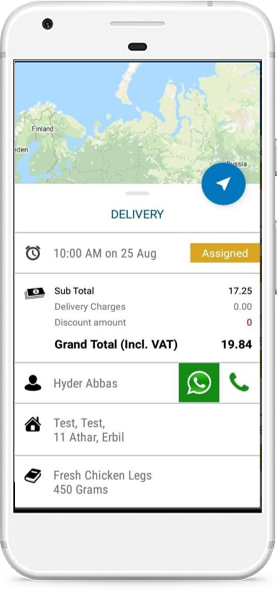The image showcases a detailed display of a white cell phone, emphasizing the functionality and layout of a delivery app. The device sports a front-facing camera dot in the top-left corner and a central speaker line. The screen, outlined by a slim black border, exhibits a user interface with various details.

At the top of the screen, a map displaying blue seas and green land is visible. Directly below the map, centered in a white block, is the word "Delivery," accompanied by a blue circle with a white arrow pointing to the top-right corner. A gray line demarcates this section from the next.

Beneath the gray line, on the left side, a clock icon is displayed, followed by the text "10 a.m. on 25 August." On the far right, an orange block with the word "Assigned" in white is present. Another gray line separates this section from the subsequent informational blocks.

The next block lists financial details: "Subtotal: $17.20", "Delivery charges: $0", and "Discount amount: $0". The "Grand total including VAT" is noted as "$19.84." 

Following another light gray line is a block on the left containing a silhouette icon of a person's head and shoulders next to the name "Haider Abbas." To the right of the name, a green block with a chat bubble and a white block with a green phone icon are visible, likely representing contact options.

Further down, another gray line precedes a house icon with the address "Test Test 11 Arthur Obel." 

The final section, demarcated by another thin gray line, lists the ordered item: "Fresh chicken legs, 450 grams."